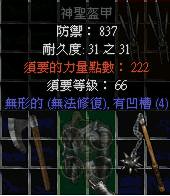The image features an ominous scene with a complex array of medieval weaponry and detailed text in Chinese. Central to the image is a figure wearing full-body metal armor, standing resolutely behind a spiked fence. The fence is standard but adorned with menacing spikes at its top. To the left of the armored figure is a sinister contraption—a tall, guillotine-like ax affixed to a wooden stack. The blade is menacing and evokes a sense of immediate danger. 

To the right, there's a piece of wood connected to a formidable spiked ball by a metal chain, resembling a deadly flail. The scene suggests that twirling this weapon could inflict devastating harm, similar to the lethal potential of the guillotine ax. Hovering above these weapons and the armored figure is an array of text primarily in Chinese, featuring colors like red, white, blue, and a greenish hue at the top. The text includes a series of numbers such as 8, 837 at the top, and 31, 31 towards the middle, with additional numbers like 2, 2, 2 in red followed by white Chinese text and then a 6, 6. 

Further down, blue Chinese text is accompanied by the number 4. The backdrop of the image is predominantly black, enhancing the foreboding and grim atmosphere. The detailed elements, from the weaponry to the multilingual text, create a rich, intricate depiction of a scene laden with historical and violent connotations.